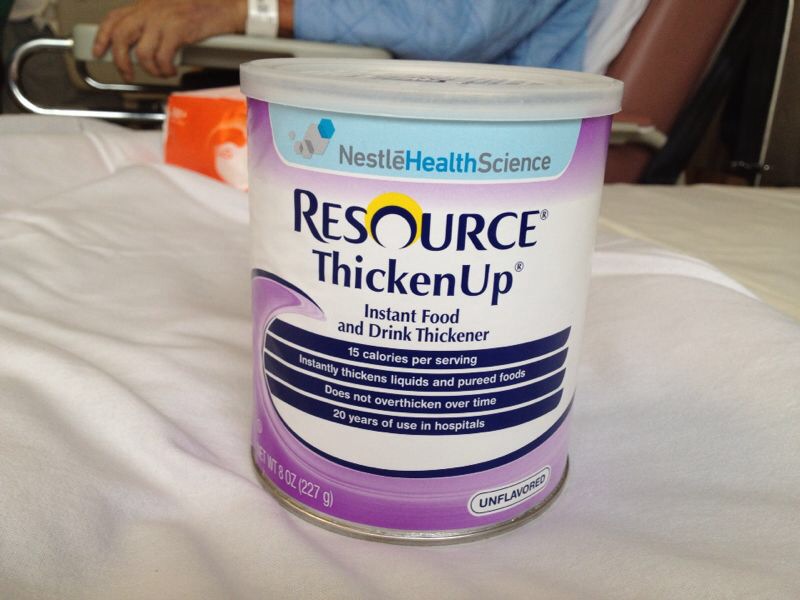This detailed image showcases a Nestlé Health Science product, specifically the 'Resource ThickenUp' Instant Food and Drink Thickener. The container is round, with a predominantly purplish-white design featuring a wave-like purple pattern. At the top of the packaging, the brand name 'Nestlé Health Science' is prominently displayed, followed by the product name 'Resource ThickenUp'. Descriptions on the label indicate that this thickener provides 15 calories per serving, instantly thickens liquids and puréed foods, and crucially does not over-thicken over time. It's highlighted that this product has been trusted for over 20 years in hospital settings. Additionally, it’s marked as 'unflavored' at the bottom, and weighs 227 grams. The container is positioned on a hospital bed, and in the background, the image shows the arm of a hospital patient donned with a hospital bracelet and gown, reinforcing the hospital setting where this product is commonly utilized.